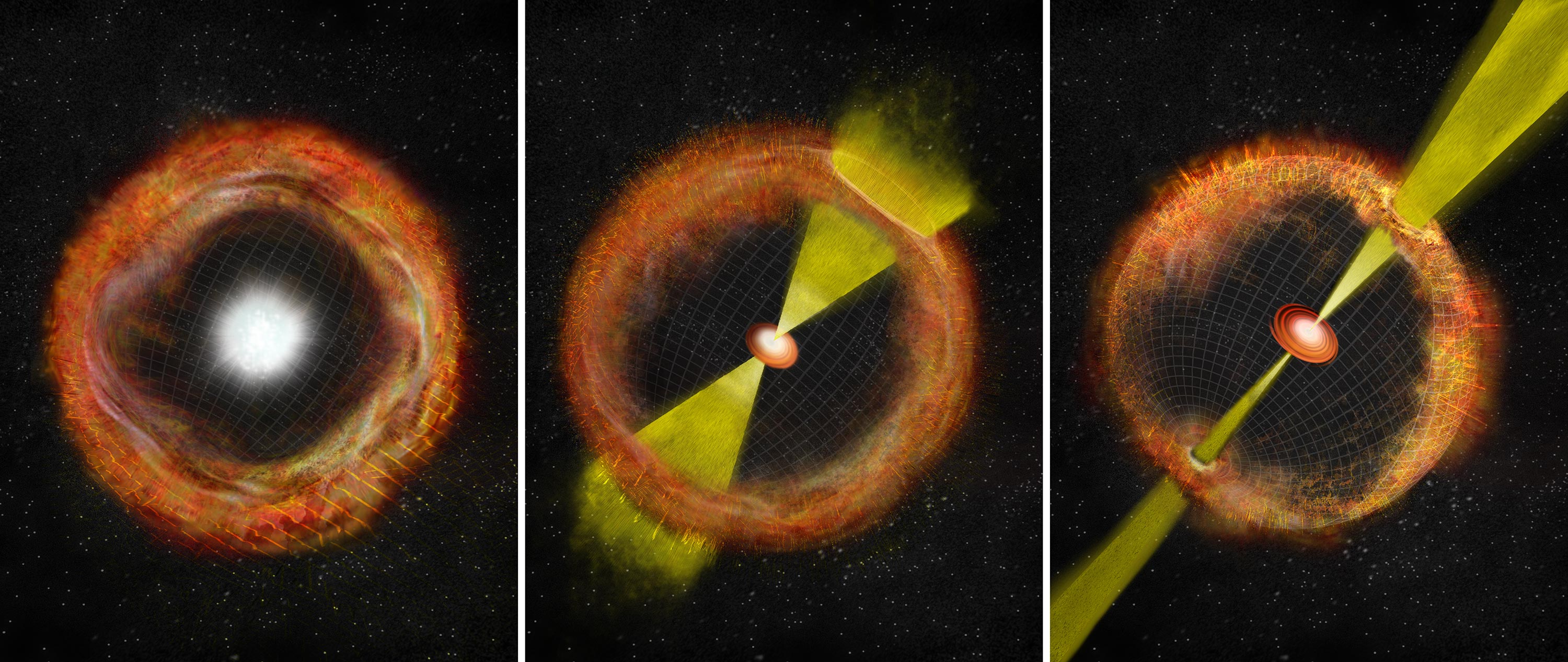This is a detailed digital illustration of a celestial event represented through three sequential images arranged horizontally. Each image depicts a similar scene, with subtle changes illustrating the progression of the event. 

In the leftmost image, a bright white sun is encircled by a dark band of open space, surrounded by a fiery ring of oranges and reds, suggesting swirling gases and cosmic activity. The background features a grid pattern, likely symbolizing the fabric of spacetime, and thin lines are seen moving across the bottom right portion of the ring.

In the middle image, the central object transforms into a circular shape with orange rings and a white core. Two cones of yellow light emanate from the white center, piercing through the surrounding red cloud. The dark band narrows, emphasizing the intensity of the central phenomenon.

In the rightmost image, the progression continues as the orange and red outer ring fragments, making the background grid pattern more distinct. The yellow cones of light are now more focused, extended, and intense, indicating an increase in energy or momentum within the celestial event.

The entire scene is set against a backdrop of dark sky with distant stars, capturing the awe-inspiring beauty and dynamism of the cosmos.